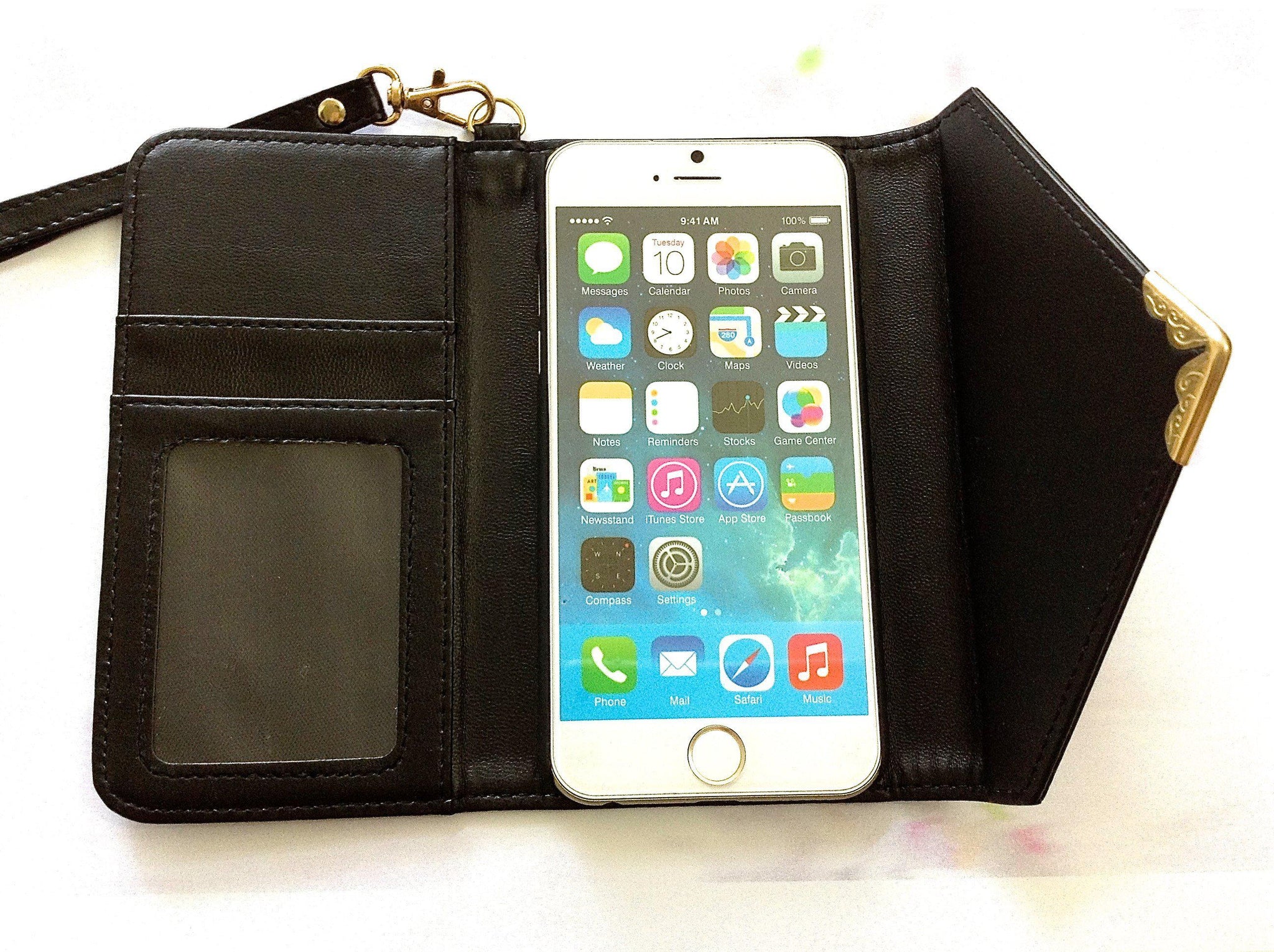The image is a detailed photograph of a black leather phone case that doubles as a wallet. The iPhone, appearing to be an older model, possibly an iPhone 6 or earlier due to the visible fingerprint function, is securely held in a lever phone holder. The case is open, showing several compartments on the left side designed for credit cards, IDs, and other papers. A transparent pocket is also visible. The phone screen, which displays multiple apps, indicates a time of 9:41 a.m., with full Wi-Fi service, five bars of cell reception, and a 100% battery charge. The apps on the home screen include Messages, Calendar, Photos, Camera, Weather, Clock, Maps, Videos, Notes, Reminders, Stocks, Game Center, Newsstand, iTunes Store, App Store, Passbook, Compass, Settings, along with Phone, Mail, Safari, and Music in the dock. The background of the photograph is predominantly white, with a faint, grainy, and blurry texture suggesting a partially erased image.